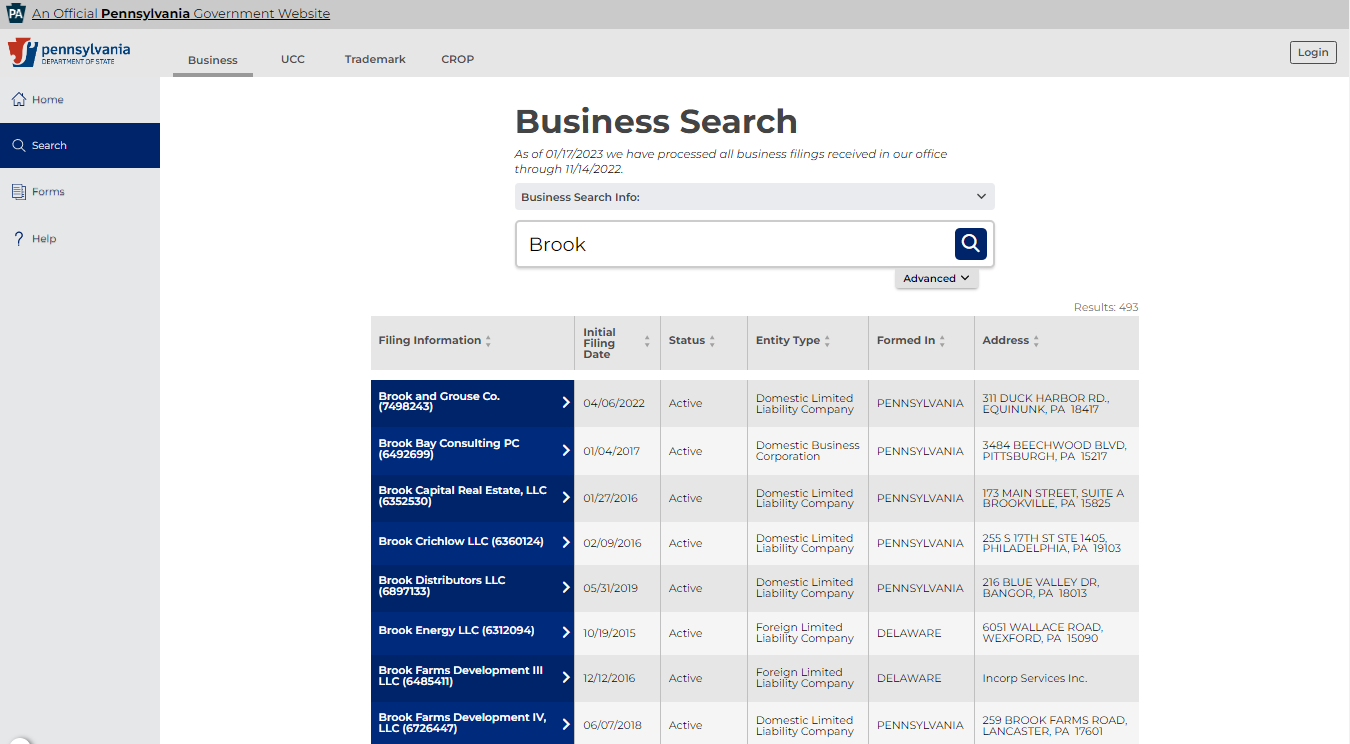This image depicts an official Pennsylvania government website interface, showcasing the structured layout specific to the Pennsylvania governmental digital environment. 

On the left-hand side of the screen, a navigation panel lists options including "Home," "Search," "Forms," and "Help." 

In the main content area of the page, several sections are visible: "Business," "UCC," "Trademarks," and "Crop." Prominently displayed is a notice stating, "As of 01-17-2023, we have processed all business filings received in our office through 11-14-2022."

A central feature of the page is the "Business Search" function, with "Baruch" entered as the search term. The search results are presented in a table format, which includes columns for "Filing Information," "Initial Filing Date," "Status," and "Entity Type, Formed In, Address."

The table lists several entities, starting with:
1. Baruch and Gross CO.
2. Baruch Bay Consulting PC.
3. Baruch Capital Real Estate LLC.
4. Baruch Creature Law LLC.
5. Baruch Distribution LLC.

The table continues beyond the visible portion, suggesting more entries related to the search term "Baruch."